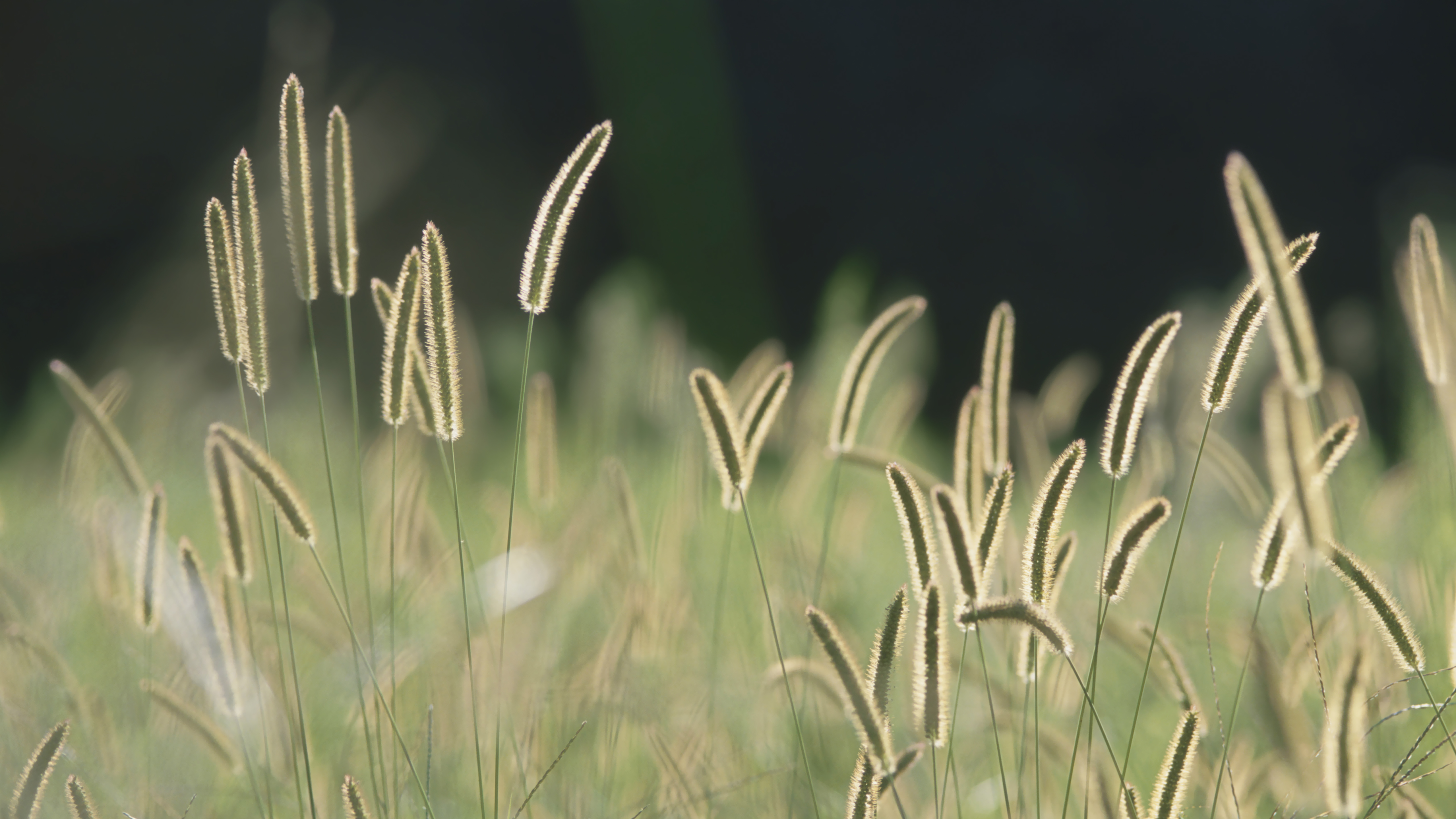This professional photograph captures a captivating outdoor environment characteristic of a prairie, focusing on wild plant life. The image centers on thin, green stems that rise sparsely from the ground, each bearing a long, fuzzy tip at the top, reminiscent of cattails. The fuzzy tops exhibit a greenish hue that appears white and beige due to the strong light illuminating the scene. The photo features a crystal-clear foreground, while the background is deliberately blurred, displaying an indistinct mix of white, yellow, and green shapes with a predominantly black upper section. This artistic use of light and focus emphasizes the stark contrast between the sharply detailed plants and the softly rendered backdrop, creating a striking visual effect.